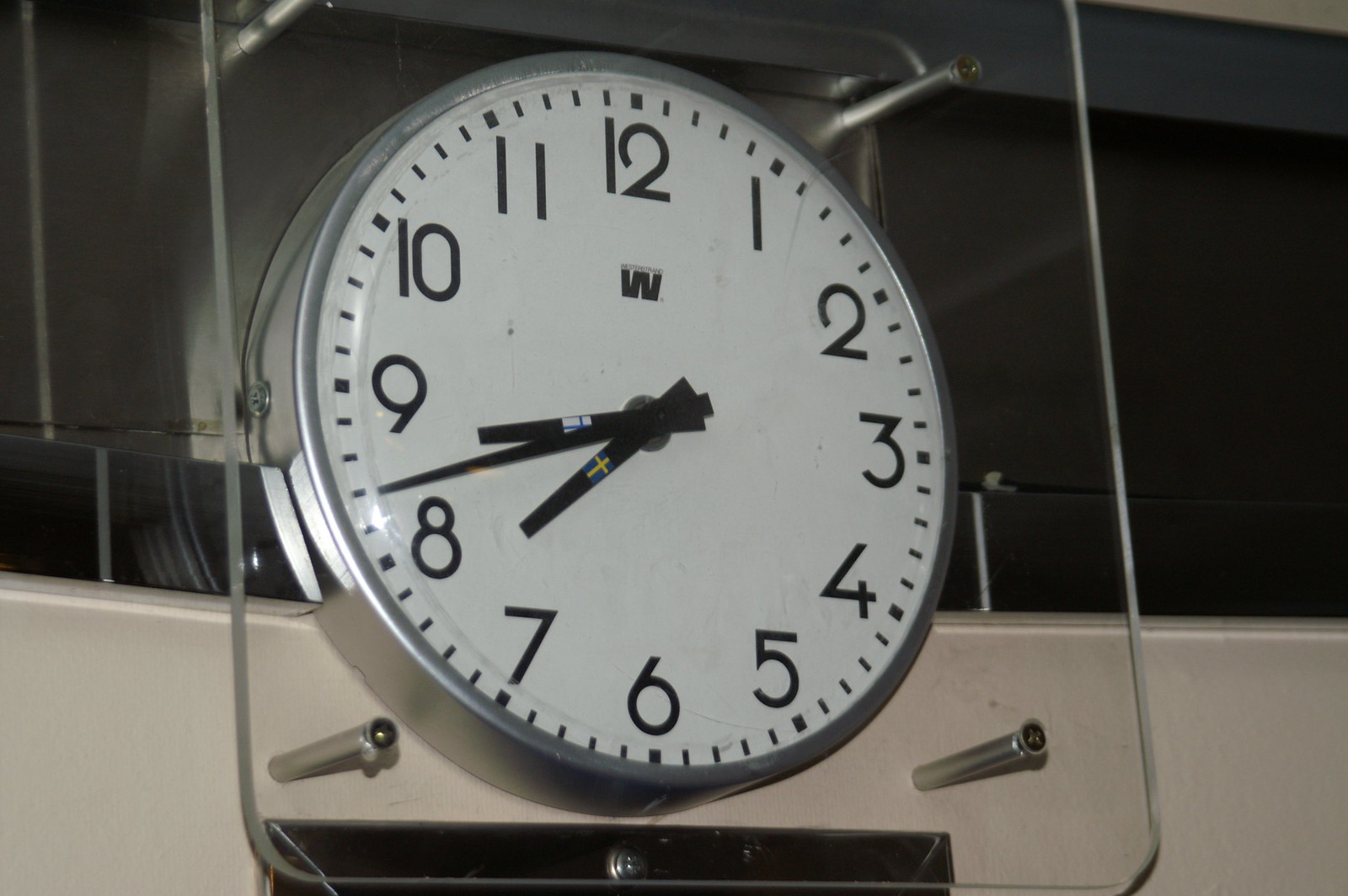This detailed photograph captures a distinctive wall-mounted clock. Encased within a sleek, silver metal frame, the round clock face is protected by a square glass panel, secured by screws into cylinder brackets. The clock’s white face is clearly visible through the glass, featuring numerals 1 through 12 arranged counterclockwise in a standard black font. The clock showcases a 'W' logo centrally located on its face. Three hands mark the time: a long, thin second hand, and two shorter, broader hands, one adorned with a pattern resembling the Swedish flag in blue and yellow and the other reflecting the Finnish flag’s blue and white design. The clock is further encased in a clear plexiglass cover, likely for protection and tampering prevention, and is fastened to a simple white wall. As captured, the clock reads 08:42.